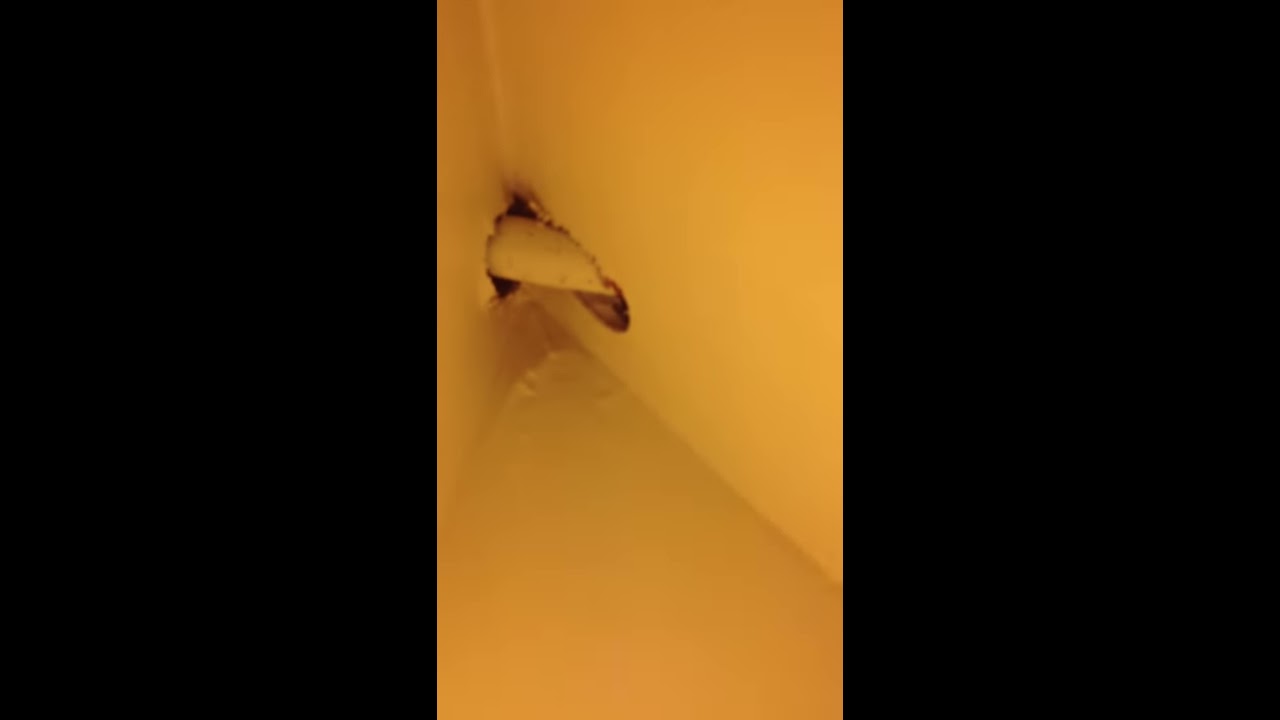The image depicts the interior of a house with a pipe protruding through a corner cutout in the drywall. The wall, painted a light cream color with a slight orange-golden cast, serves as the backdrop. The center area, specifically a 9x16 portrait orientation, features this protruding pipe. Flanking the center image are two black rectangles on either side, framing the central scene. The photo shows the pipe extending through two holes positioned near a seam where two walls meet, suggesting a connection or continuation through the wall. There are no visible people, buildings, vehicles, or text, giving full focus to this structural detail. The image's composition and the way it's framed hint at cropping from a smartphone video or social media platform like YouTube, Instagram, Facebook, or TikTok.